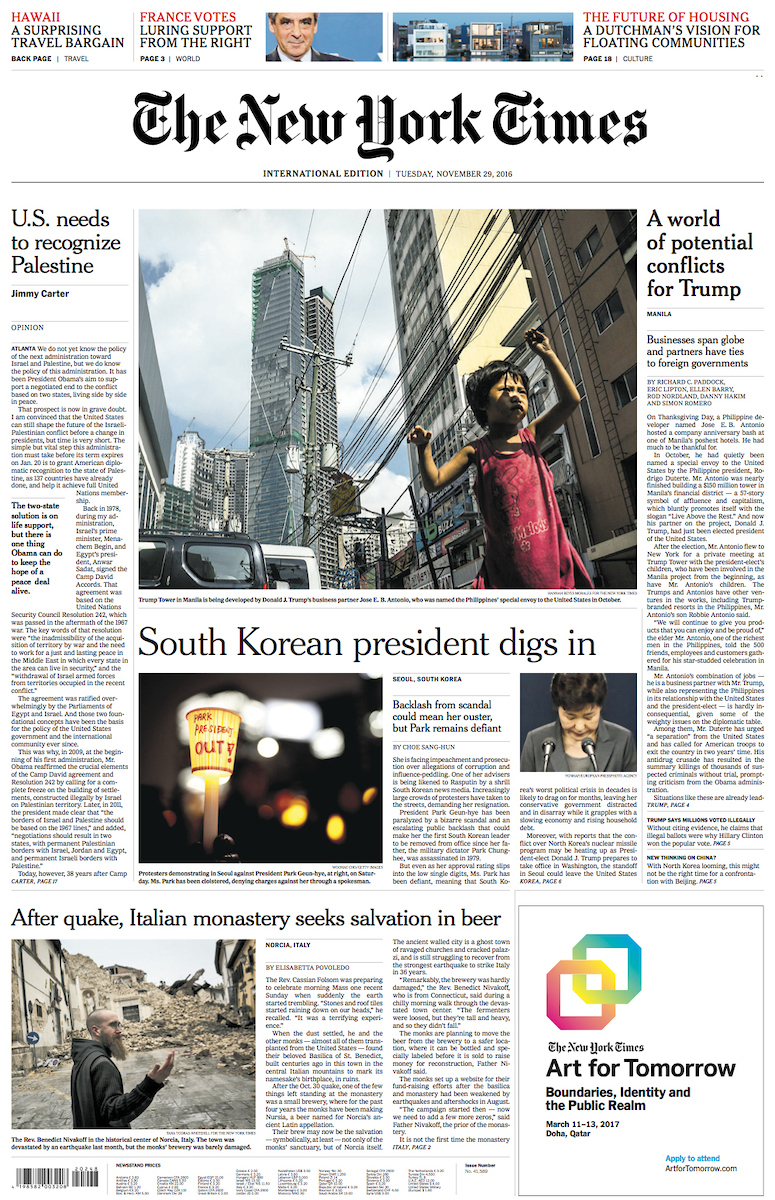A detailed New York Times cover is prominently displayed, dominated by several diverse headlines and images. 

At the top, a red headline reads "Hawaii," followed by the subheading "A Surprising Travel Bargain" in black text, hinting at enticing vacation opportunities. Below this, another red headline states "France," with the accompanying black subheading "Boats Luring Support from the Right," suggesting a political piece. 

The cover also features an image of a light-skinned man, partially visible in a suit, beside another photograph depicting a cluster of houses in white and gray hues. Nearby, a red headline announces "The Future of Housing," with the black subheading "A Dutchman’s Vision for Floating Communities," indicating a story about innovative urban planning.

Centrally placed in large, bold black font is the title "The New York Times." Below it, a headline asserts "U.S. Needs to Recognize Palestine," adjacent to an image of a cityscape. In the foreground, a child dressed in red, with black hair, grips a black wire, adding a human element to the geopolitical discussion.

Another headline, "A World of Potential Conflicts for Trump," addresses global issues, while "South Korean President Digs In" features a person with black hair and dressed in gray, speaking into a microphone.

Further down, an article discusses the aftermath of a quake, highlighted by the headline "After Quake, Italian Monastery Seeks Salvation in Beer," accompanied by an image showing building rubble and a bearded individual in a hoodie.

Additionally, an image of a hand holding a candle, partially silhouetted by a Dixie cup, accompanies another article, adding a touch of human resilience.

Lastly, an advertisement at the bottom promotes an art event with the caption "The New York Times Art for Tomorrow: Boundaries and Identity in the Public Realm," illustrated by two interlocking colorful circles, one in green and blue, the other in pink and yellow.

Overall, the cover offers a rich tapestry of stories, each accompanied by compelling visuals and headlines, catering to a wide array of reader interests.